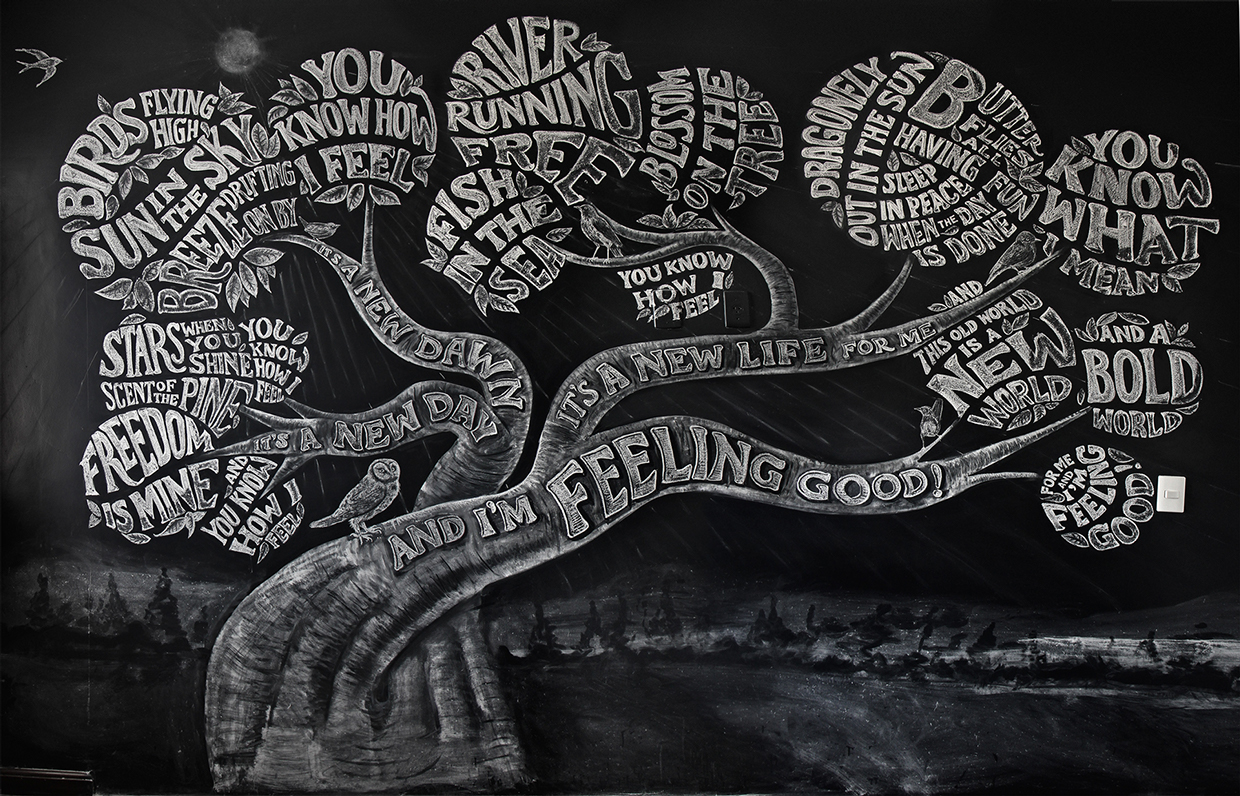The black-and-white image is a striking visual representation of a large tree that dominates approximately 75-80% of the frame, set against a dark, nighttime background with subtle tree shadows. Intriguingly, the tree is composed entirely of song lyrics, specifically from Michael Bublé's rendition of "Feeling Good." The trunk, wide and slightly split, prominently features phrases like "I'm feeling good." Its branches further extend with words and phrases such as “Birds flying high, sun in the sky, breeze drifting on by, you know how I feel,” and “Fish in the sea, river running free, blossom on the tree, you know how I feel. It's a new life, it's a new dawn, it's a new day and I'm feeling good." Additional text on the branches includes, "This old world is a new world," "freedom is mine," and "you know what I mean." Nestled on one of the branches is an owl, adding an element of nocturnal mystery to the artwork, which is meticulously filled with evocative lyrics and phrases, creating a captivating interweaving of nature and song.